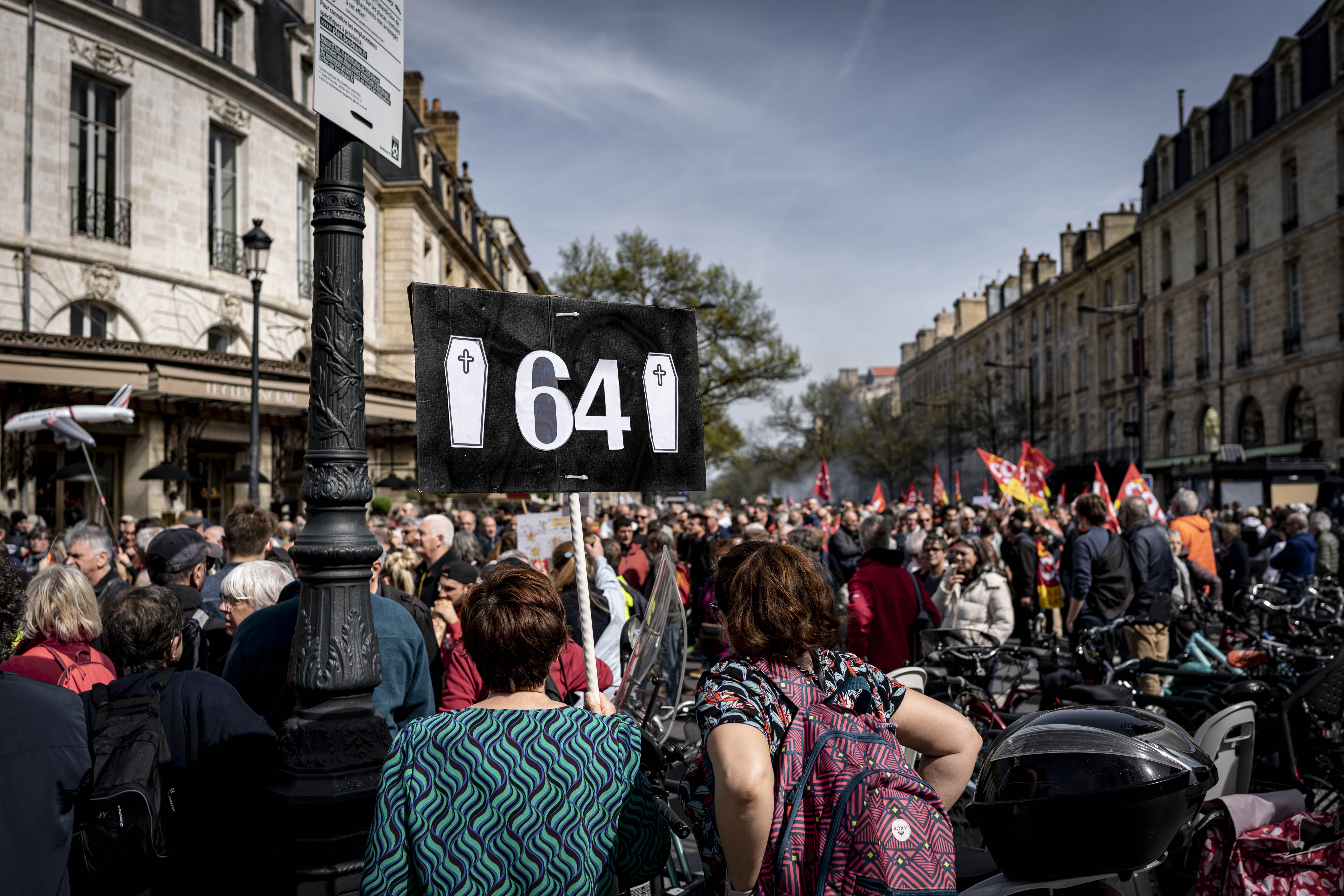This color photograph captures a large protest taking place on a crowded street in France. The image, likely taken by another protester, is in landscape orientation and vividly details the throng of people filling the entire street. The protest is marked by a sea of red and yellow flags, and there is a noticeable cloud of white smoke hanging over the distant part of the crowd. 

In the foreground, two women stand with their backs to the viewer. The woman on the left, dressed in a green dress, is holding a black rectangular sign high above her head. The sign prominently features the number 64 in white text, flanked by two white coffins, each with a black cross. Beside her, another woman carries a paisley-looking backpack. 

The street is flanked by rows of older, off-white brick buildings with dormer windows gracing their flat roofs. These structures are generally three to four stories high and add a sense of historical context to the scene. A black metal light pole and a couple of green trees punctuate the urban landscape. The sky above is a mix of blue and clouds, providing a moody backdrop to this moment of civic expression.